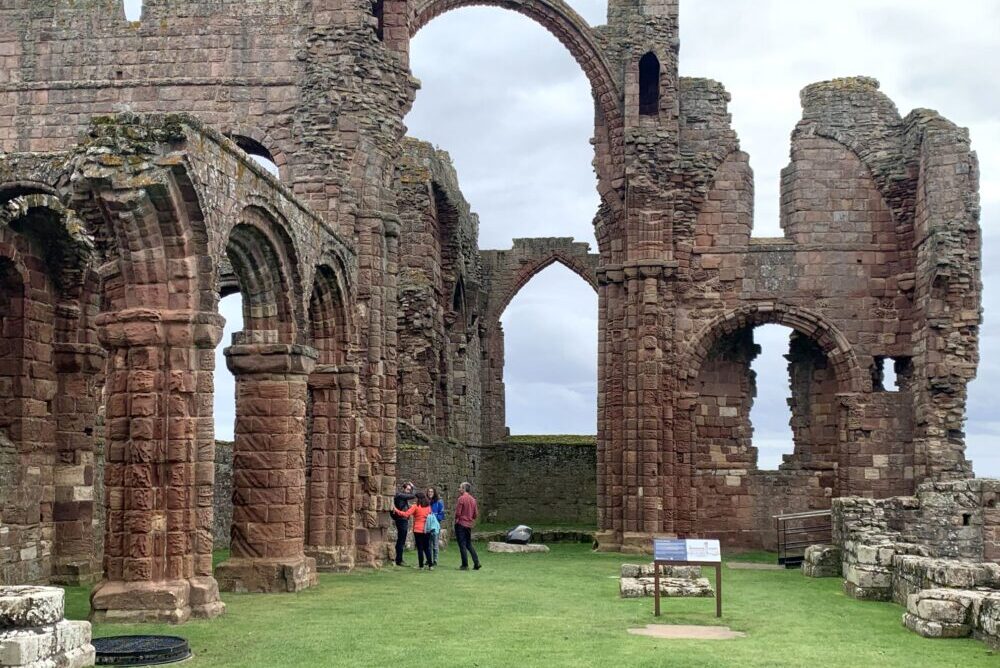The image depicts the ancient ruins of the Lumia Cultural Heritage Site, reminiscent of a dilapidated castle or possibly a cathedral, with striking similarities to St. Andrews in Scotland. The weather is agreeable—clear skies with a hint of overcast—casting an even light on the scene. The focal point is the aged structure, constructed predominantly from red and brown bricks, many of which are now decayed and covered in patches of moss. The edifice features numerous arches and circular elements, contributing to its historical charm. On the far left, two towering pillars with arches draw the viewer's eye. Towards the middle of the image, a blue-and-white informational sign hints at the site's storied past. The lush, green grass surrounding the ruins adds a vibrant contrast to the earthy tones of the bricks. In the central area, a small group of four people can be seen; one woman touches the weathered walls, while others, potentially tourists, listen to what appears to be a tour guide. Their presence adds a human element to the scene, emphasizing the cultural and historical significance of the site.